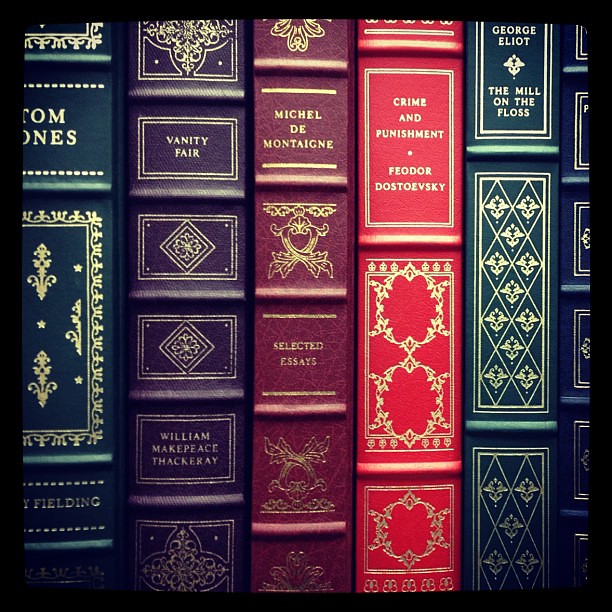This image showcases a close-up of several book spines neatly lined up on a shelf, highlighting their elegant and regal appearance. The spines exhibit traditional gold etchings with symbols and titles that suggest literary classics. From left to right, the spines display various colors: a dark blue book with the partially visible author "Fielding" on its spine; a purple book with "Vanity Fair" by William Makepeace Thackeray; a violet or lighter purple book, also featuring grand golden designs; a bright red book for "Selected Essays" by Michael de Montaigne; a dark green book with "George Eliot" and a possible title "The Mill on the Floss"; and finally, another dark blue book, though only a small portion of its spine is visible. The books' gold inscriptions appear delicate and carefully crafted, adding to their distinguished old-school charm.